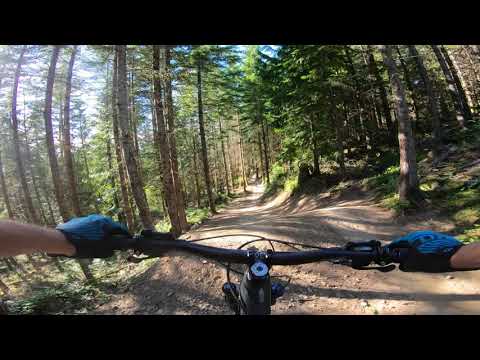In the image, captured from the first-person view of someone riding a mountain bike, you can see the handlebars of the bike prominently in the foreground. The rider, who has bare arms and white skin, is wearing distinctive blue gloves with black-colored insides. The bike's handlebars are thin and feature a small blue circle where the sides converge, with a slight glimpse of the wheel below. The path ahead is gravelly and dirt-covered, marked with rocky patches, and appears to be descending a mountain. On either side of the pathway, tall coniferous trees create a natural corridor; the trees on the left are particularly towering, with trunks rising from the bottom to the top of the image, while the trees on the right display more visible leaves and less trunk. The scene is lit by sunlight originating from the left, casting shadows onto the road. The image has a concave, slightly distorted appearance due to the use of a GoPro-like camera, affixed possibly on the rider’s helmet, complete with black letterboxing bars at the top and bottom, further emphasizing the intense perspective of the downhill ride amid the trees.